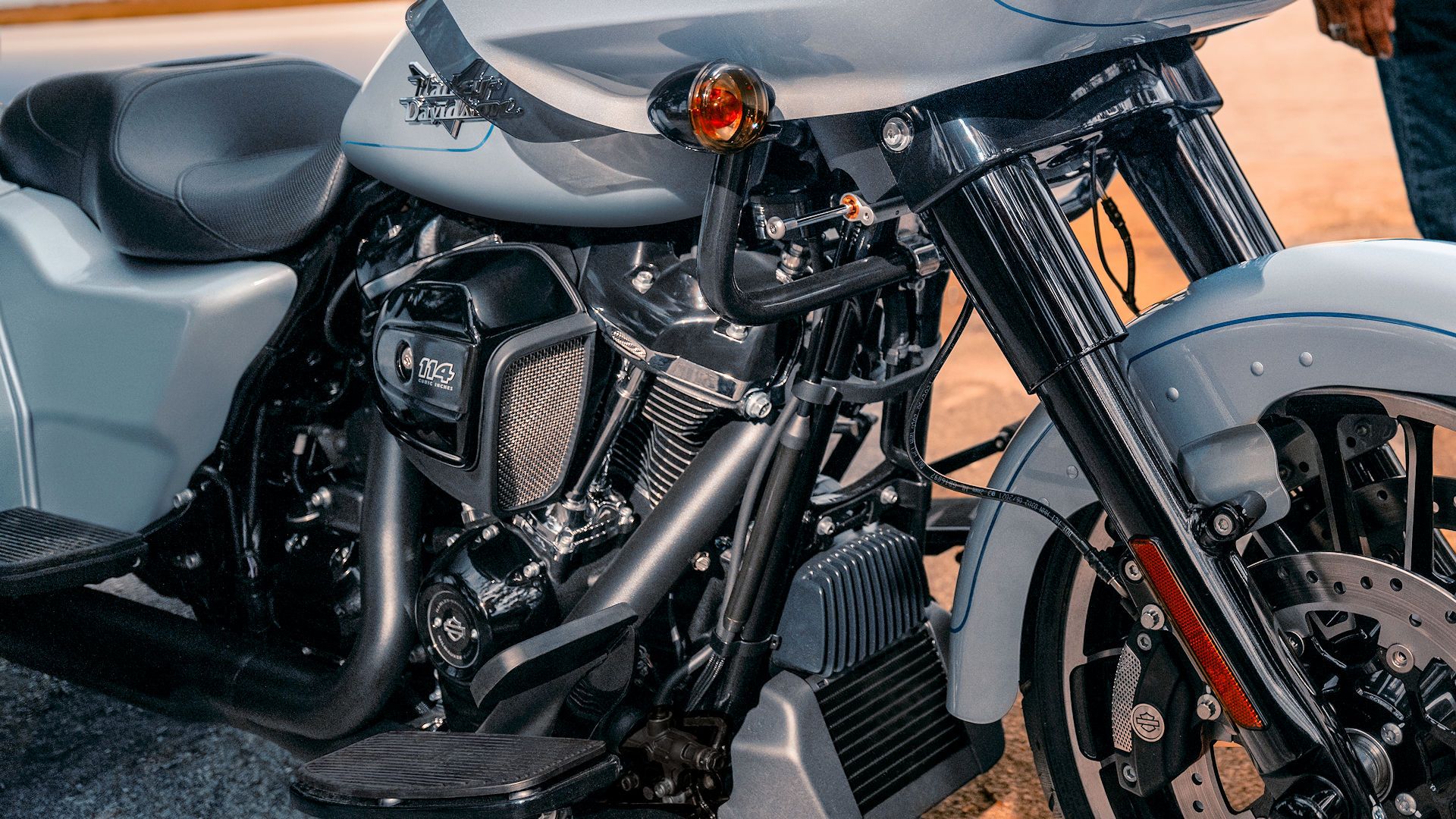The photo features a Harley-Davidson trike motorcycle, predominantly showcasing its metallic gray and black color scheme. The finish on the gas tank is particularly glistening, with a shiny, light gray to metallic hue that contrasts with its numerous black components, such as the foot pedals and shock absorbers. The front wheel is clearly visible, featuring black spokes and silver rims, and the motor prominently displays "114 cc". Reflector lights and red headlights add vibrant touches to the otherwise monochromatic design. The engine block, also black, is partially visible, indicating it’s a newer model. In the top right corner of the image, a person’s hand and leg clad in blue jeans can be seen, adding a human element to the scene. The background appears slightly blurred, resembling a dry, desert-like terrain, which further emphasizes the motorcycle as the focal point.